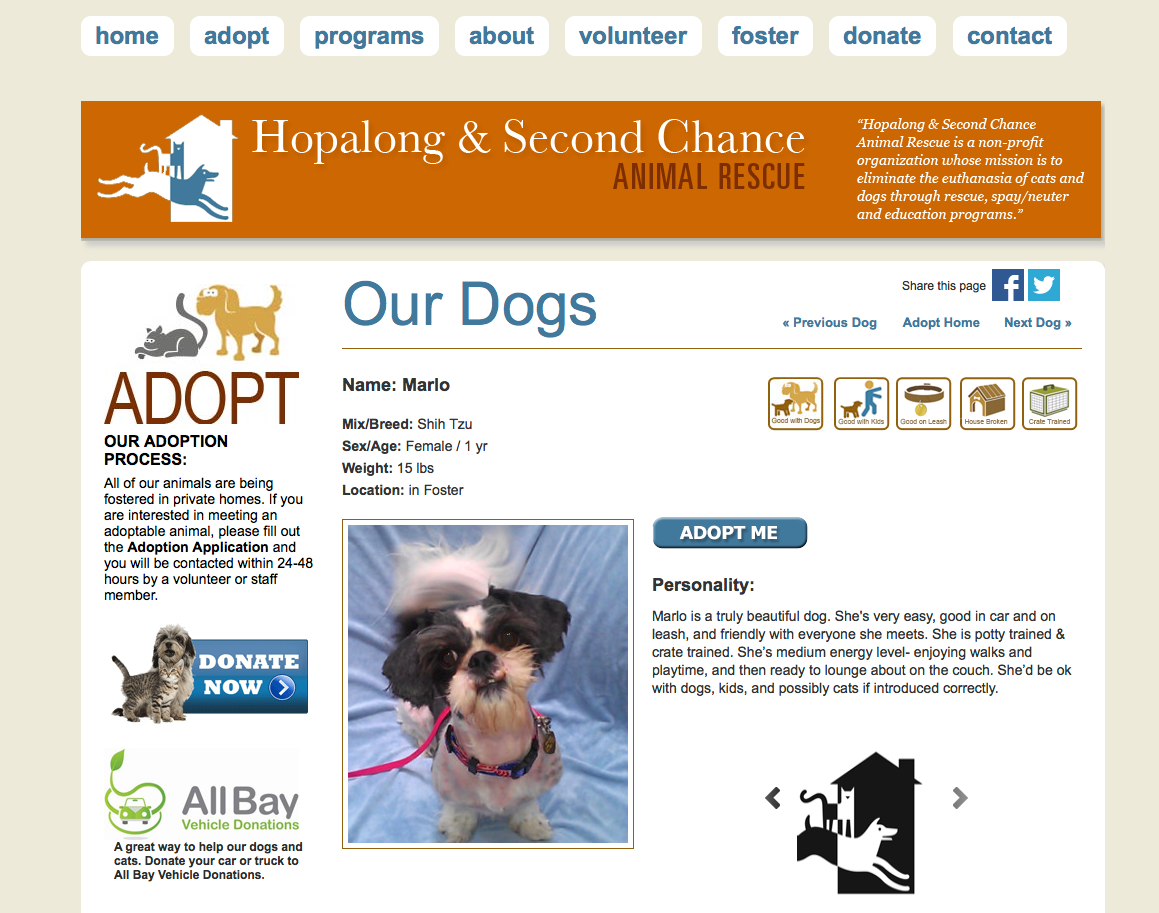This page belongs to the Hop Along and Second Chance Animal Rescue Society and provides detailed information about their dogs and the adoption process. Featured prominently is Marlo, a one-year-old female Shih Tzu weighing 15 pounds, currently staying in foster care. Marlo is described as a truly beautiful dog who is very easy-going, both in cars and on a leash, and friendly with everyone she meets. She is potty trained and crate trained, and exhibits a medium energy level, enjoying walks and playtime but also appreciating downtime on the couch. Marlo is comfortable with dogs, kids, and possibly cats if introduced correctly.

Additionally, the page features a "Donate Now" button along with a picture of another dog and a cat. It promotes All Bay Vehicle Donations as a great way to support the rescue's animals. The organization encourages people to donate their cars or trucks to assist in the rescue efforts.